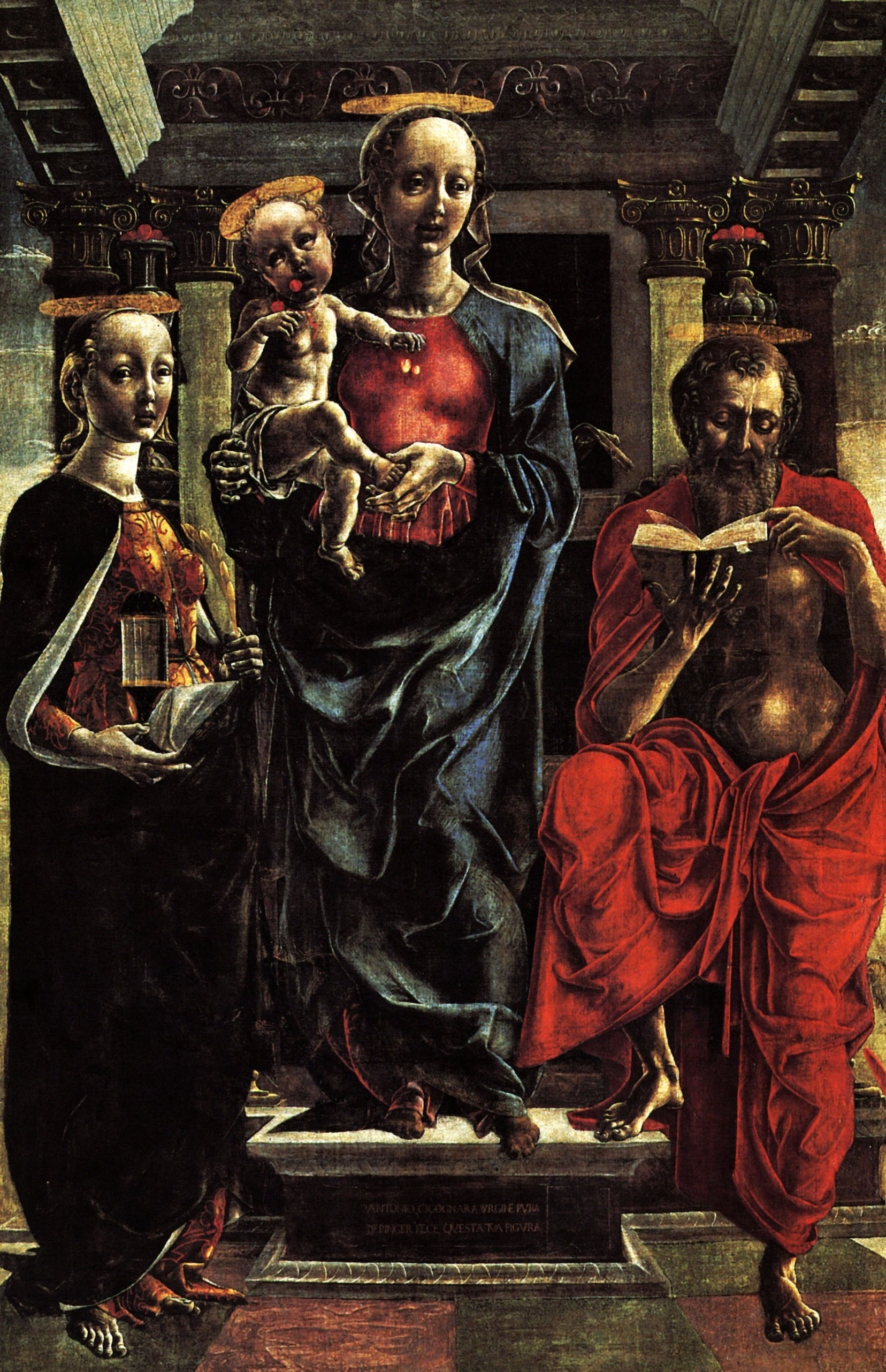In this detailed painting, we see a scene featuring four figures with an air of mystique. On the far right, a bearded man dressed in a long red robe is absorbed in reading a book he holds in one hand. His attire is complemented by a metallic sheen, common across the figures. To his left stands a woman in a long black robe with a metallic object on her chest, suggestive of an eerie ambiance. Centrally positioned, another woman dressed in a blue robe is cradling a baby with just a cloth around its bottom and reddish hair. The group exudes an angelic aura, each adorned with metallic halos casting a golden glow. They appear to be in a grand hall or castle, featuring ornate woodwork and a checkered black and red tiled floor. The podium and towering pillars further enhance the scene's regal and somewhat otherworldly atmosphere.